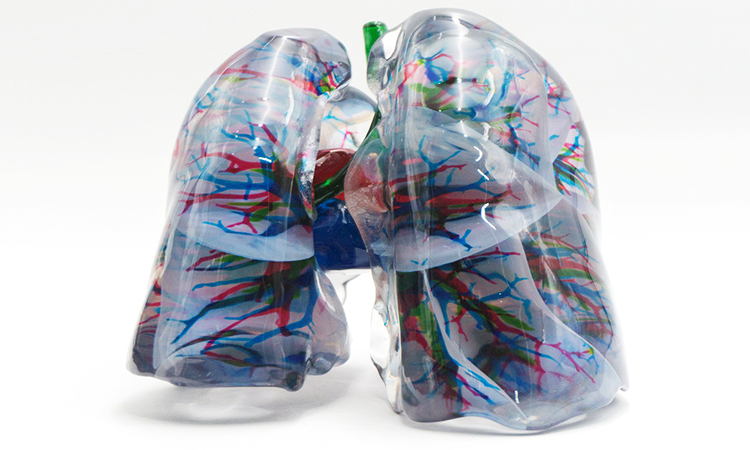The image features an abstract, colorful model resembling a pair of human lungs crafted from shiny, transparent plastic. The central structure is composed of two lung-shaped sections with intricate red and blue squiggly lines running through them, mimicking veins and arteries. These vibrant lines are embedded in the clear plastic, creating an effect reminiscent of blood circulation. At the core and slightly to one side of the model, there are more solid patches of red and black, interspersed with green, possibly representing a deeper anatomical structure. Radiating behind this core, deeper blue and red elements add complexity to the design. The plastic material is reflective, giving the entire piece a striking, glossy appearance. It appears as an abstract decorative object, merging elements of anatomical illustration and modern art.